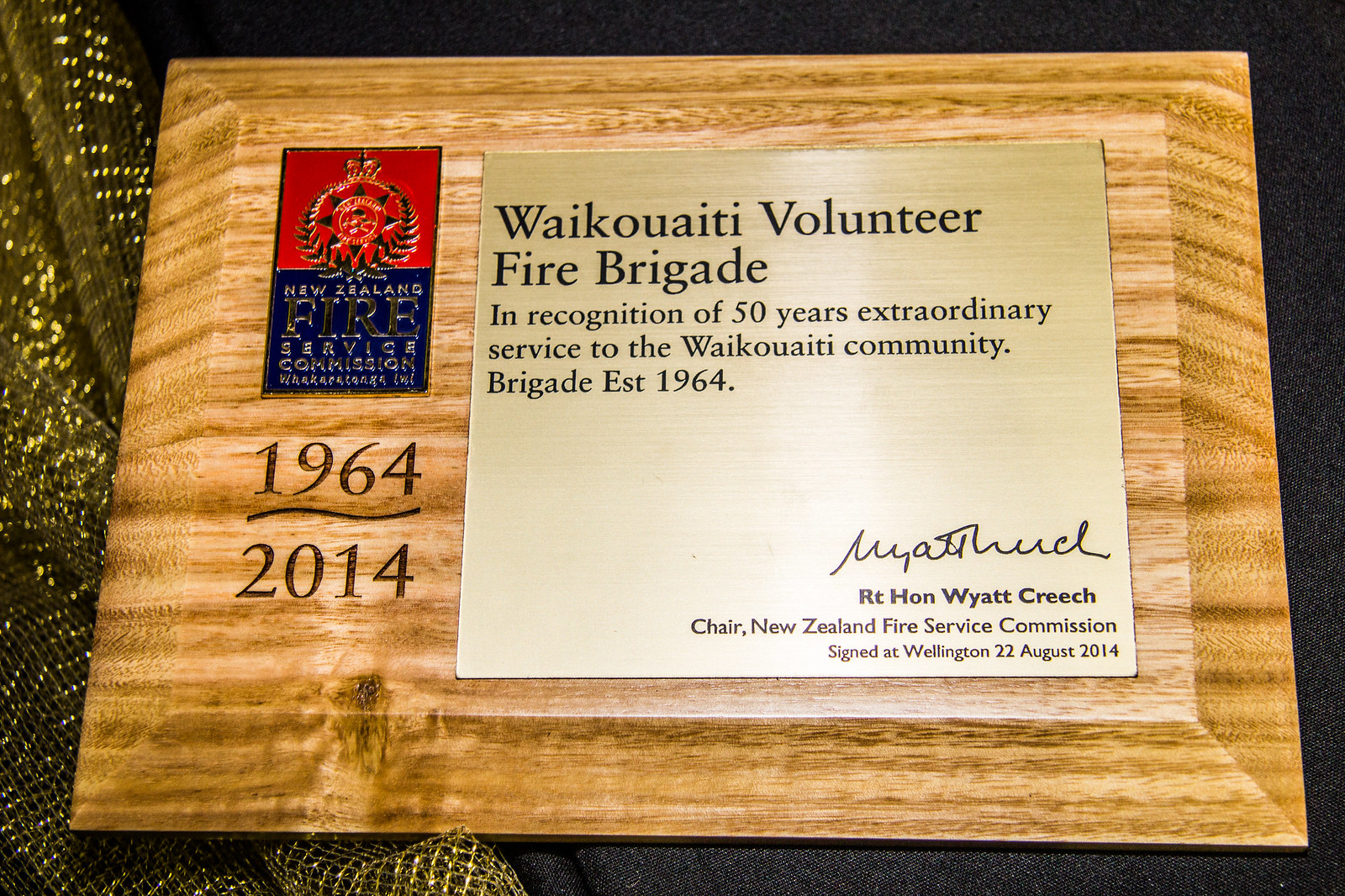This image features a wood-grain plaque set against a predominantly black background, with a sparkly and mushy texture on the left side. The plaque, made from lighter wood with darker green hues blending from left to right, prominently displays the dedication and service of the Waikoua'ati Volunteer Fire Brigade. 

In the top left corner, there's a vertically rectangular logo divided into two sections: a red upper half with an emblem and a blue lower half bearing the inscription "New Zealand Fire Service Commission". Beneath this logo, etched directly into the wood, are the years "1964" and "2014" separated by a line. To the right, a gold-colored square plaque is affixed, engraved with the following details in black letters: "Waikoua'ati Volunteer Fire Brigade in recognition of 50 years of extraordinary service to the Waikoua'ati Community. Brigade established 1964."

The bottom right corner of the gold plaque features a signature followed by the designation, "Retired Honorable Wyatt Creech, Chair, New Zealand Fire Service Commission," along with the signing details, "Signed at Wellington, 22 August 2014." A subtle golden ribbon or ribbon-like texture is also visible underneath the plaque on the left-hand side.